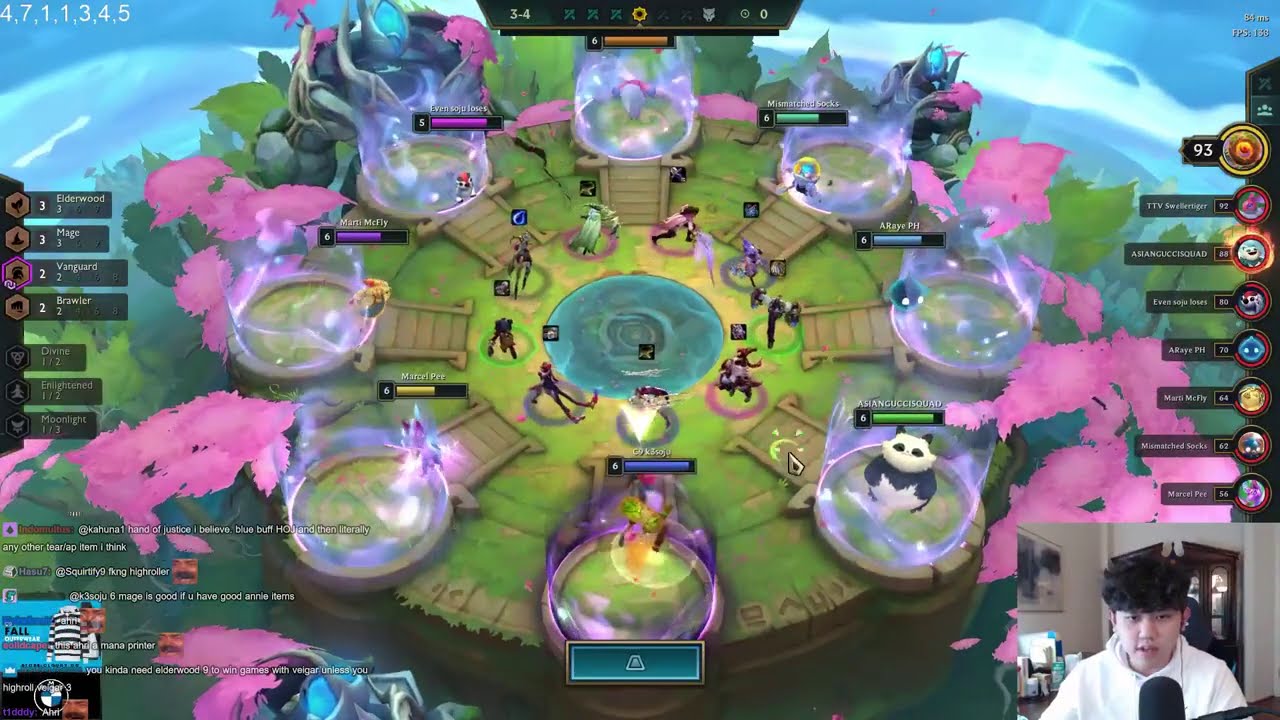This screenshot captures a young Asian man playing a colorful animated video game on his computer or television. In the bottom right corner, an inset live webcam view shows him wearing a white hoodie and sitting in front of a large black microphone. The background of his room includes a brown china cabinet against the wall and a shelf with various products, suggesting it's a bedroom.

The main game screen is set in a vibrant forest environment characterized by green grass, brightly colored pink leaves, and a violet haze. The forest seems encircled by a body of blue water. Multiple round spheres appear throughout the scene, some filled with glowing fairy dust and others featuring characters like a panda bear, a witch, and an elephant. These characters appear to be part of a multiplayer game, possibly engaged in battle. The outer circle of characters has life bars or power meters that go up to six, and some characters seem to be fighting without a protective force field. The game interface includes round icons with black labels on both the left and right sides of the screen.